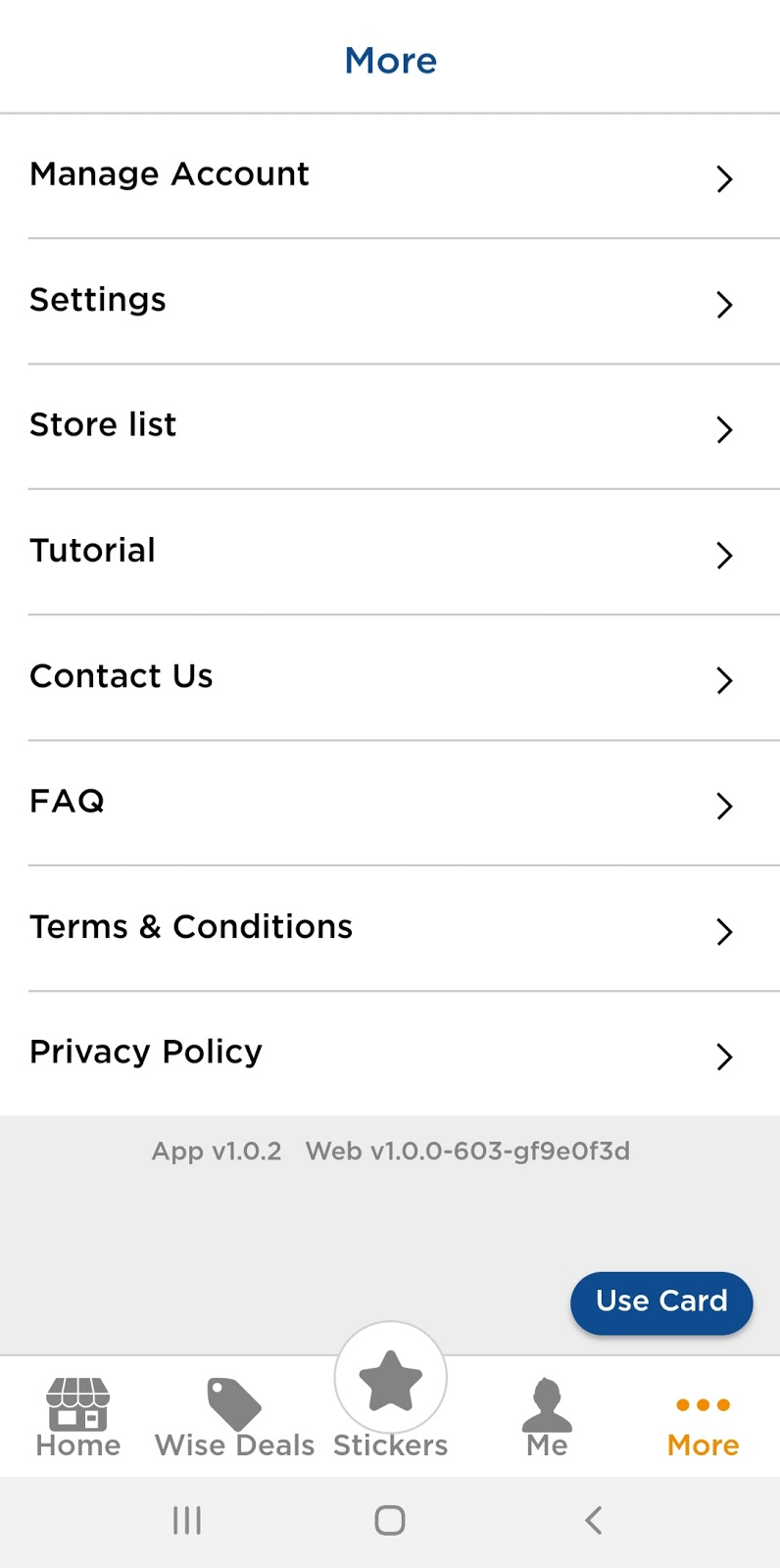This is a vertically-oriented screenshot of a webpage centered on the screen, featuring a white background segmented by thin gray horizontal lines. At the top, the header displays the word "More." Running vertically down the left-hand side of the page, between the horizontal separations, are the menu items: Manage Account, Settings, Store List, Tutorial, Contact Us, FAQ, Terms and Conditions, and Privacy Policy. At the bottom, there's a gray horizontal section with technical details that read: "App Version 1.0.2, Web Version 1.0.0-603-GF9E0F3D." On the right side of this section is a prominent blue oval-shaped button labeled "Use Card." Stretching across the very bottom of the screen are navigation icons labeled Home, Wise Deals, Stickers, Me, and More.